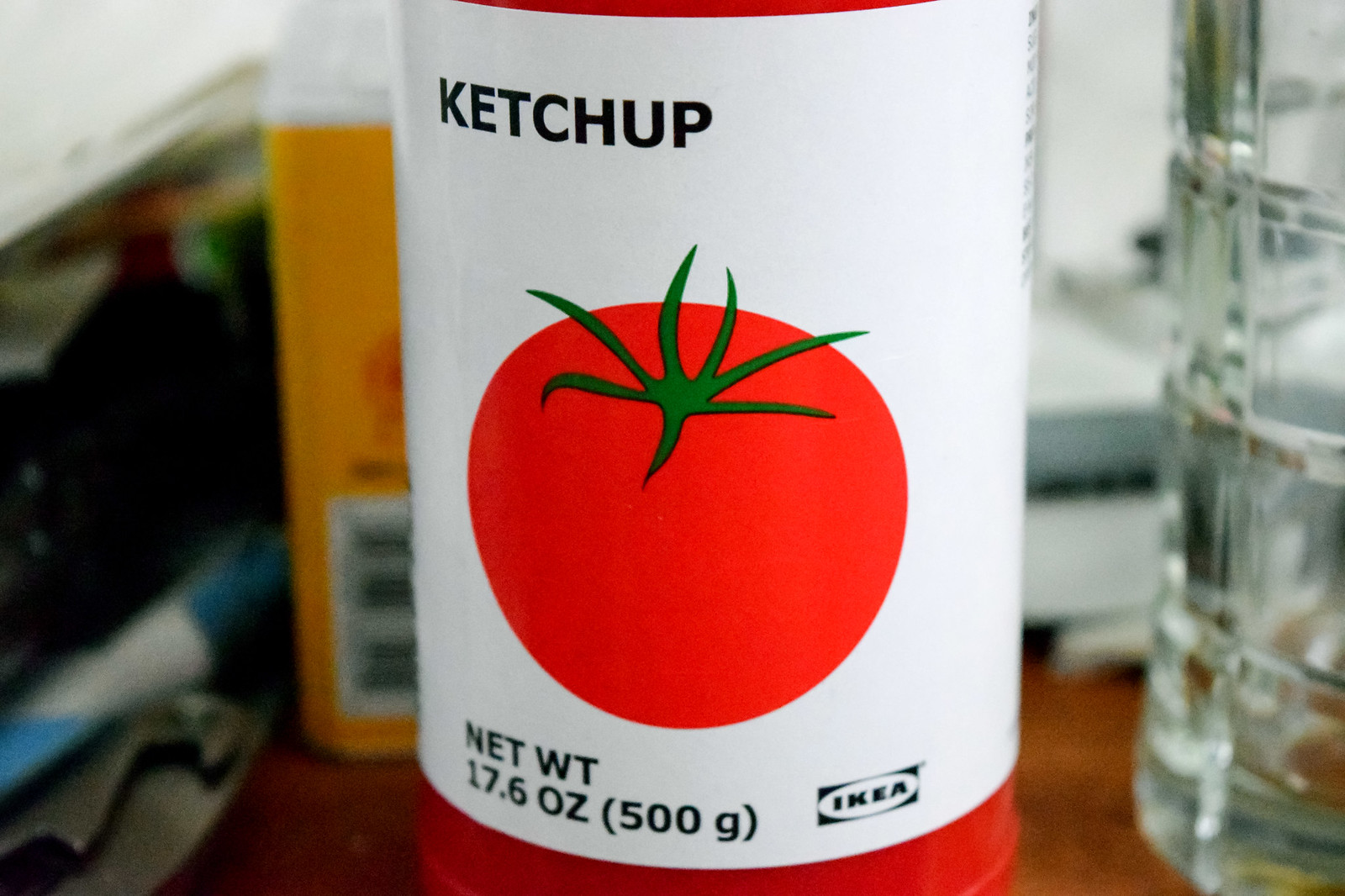The image is an up-close shot of a bright red, cylindrical ketchup bottle, prominently placed in the center, with a white label wrapped around it. The label is minimalistic, featuring "ketchup" printed in black at the top. In the middle, there is a large, round red tomato with seven green leaves sprouting from the top in a clockwise direction. Below the tomato, the label displays "NET WT. 17.6 OZ (500 G)" in black print. On the bottom right, the IKEA logo is clearly visible. The bottle sits on a brown table, under bright lighting, which contrasts with the darker, shadowy background. To the right of the ketchup bottle, there is a slightly visible glass container with etched lines, containing a small amount of an unspecified beverage. Also to the right, a yellow container with a white top and a QR code is partially seen, blurry and indistinct. The backdrop includes a blurry white wall, what appears to be a stack of white books, a blue-and-white pin, some possible metal objects, and out-of-focus bottles and fabric folds, making the setting appear cluttered and varied in texture and color.